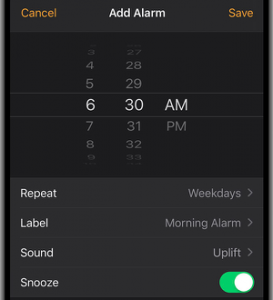Screenshot of a phone's alarm setting interface with a black background. At the top left corner, "Cancel" is written in orange text, and at the top right corner, "Save" is in the same orange hue. Centered between these two options is the white text "Add Alarm." Below the header, there are two columns of digits: the left column lists hours from 1 to 12, and the right column lists minutes from 1 to 59. Additionally, there are AM and PM sections for setting the time. The current alarm is set to 6:30 AM. 

Beneath the time setting, a configuration box with four rows is displayed. The first row is labeled "Repeat: Weekdays," indicating that the alarm will only go off on weekdays. The second row is "Label: Morning Alarm," specifying the name of the alarm. The third row is "Sound: Uplift," indicating the chosen alarm tone. The final row is "Snooze," toggled on with a green switch, enabling the snooze function. All text, except for "Cancel" and "Save," is displayed in white.